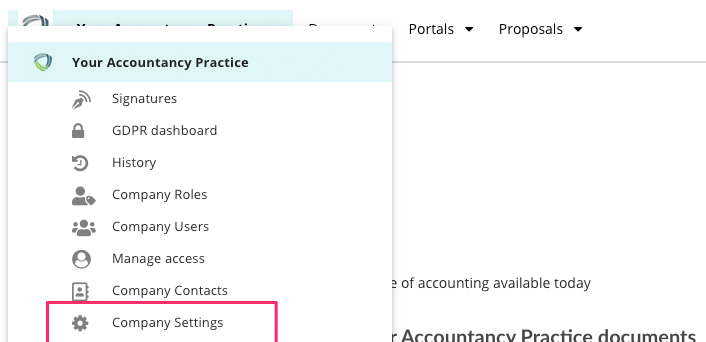This detailed caption is formulated based on the initial voice-given description:

The image showcases a user interface screen featuring various elements related to company management and settings. At the top of the screen, there is a navigation bar with several tabs labeled: "Your Accountability," "Practice," "Signatures," "GDPR Dashboard," "History," "Company Roles," and "Company Users." To the far right of the navigation bar, there is a small human icon representing user accounts, followed by a "Manage Access" button and a "Company Contacts" button. 

One of the tabs, "Company Settings," is highlighted, indicating it is the currently selected view. Adjacent to this highlighted tab is a small gear icon, suggesting it is related to settings or configurations.

Beneath the tabs, there is a prominent long red line, visually separating the top navigation from the content below.

Within the content area, there is a section where a pop-up partially obstructs the view. Despite the obstruction, some text is visible which reads: "...of accounting available today. Accountancy practice documents."

Above this, there are additional tabs, including "Portals" and "Proposals," suggesting different areas of functionality offered by the interface.

Overall, the interface appears to be part of a comprehensive dashboard designed for managing various aspects of an accountancy practice, including user roles, access settings, and important documents.